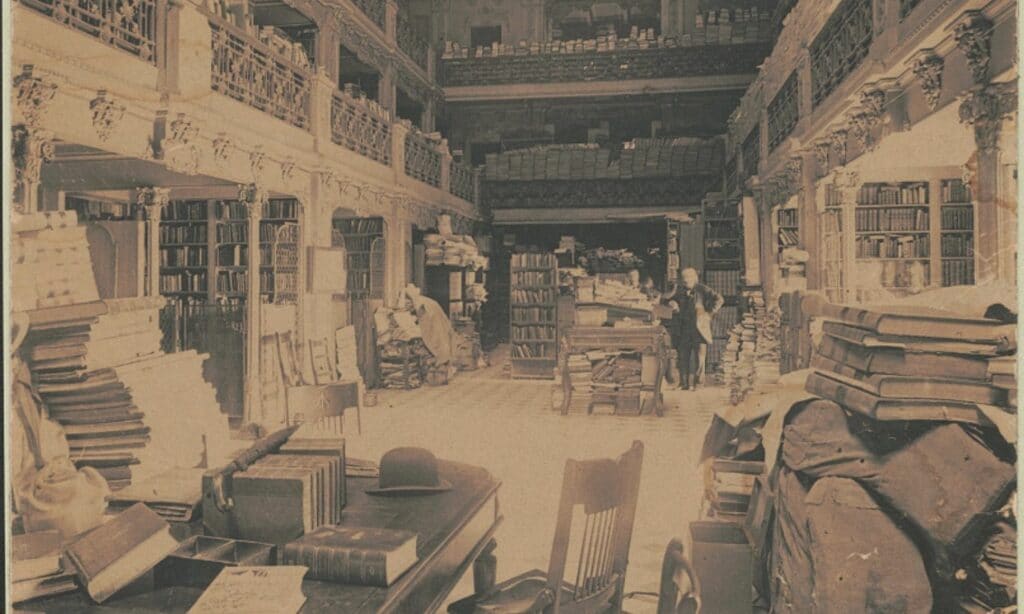The image captures an expansive, historic library showcasing a grand, elegant design supported by robust stone pillars on both the lower and upper levels. Towering bookshelves line the walls, extending up to the second floor, creating a labyrinth of literary works. Central to the scene, numerous books are scattered and stacked atop tables, while others form precarious piles beneath them. A simple wooden chair is placed prominently in the foreground, hinting at a place for quiet study amidst the chaos. In the mid-background, a man dressed in a formal black suit leans casually against a counter or bookshelf, intently gazing at the heap of books that dominate the center of the image, adding a touch of human curiosity to the scholarly ambiance.